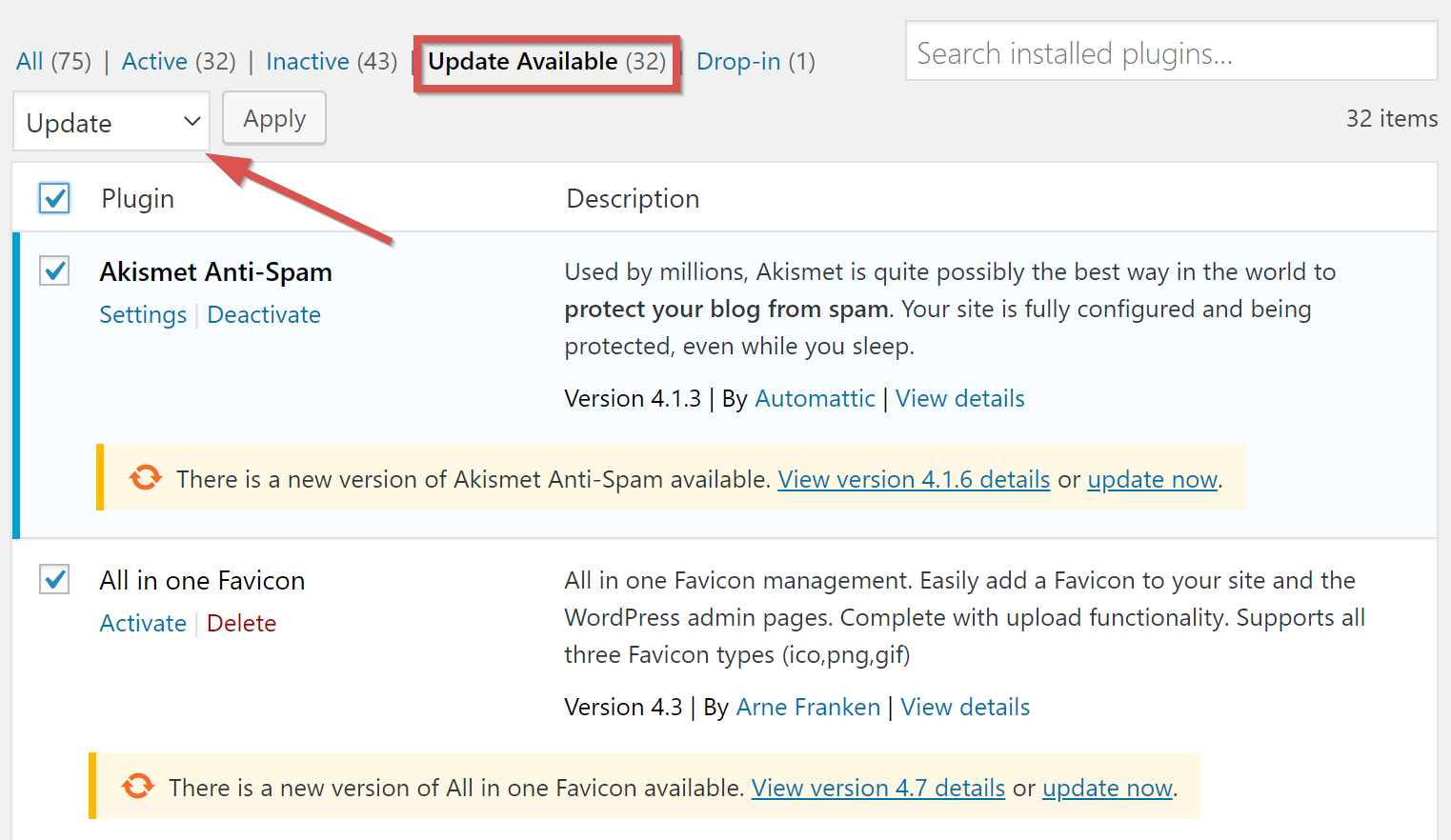The image showcases a light blue background displaying a plugin management interface for a website. 

At the top, it presents various plugin metrics:
- Total plugins: 75
- Active plugins: 32
- Inactive plugins: 43

Beneath this, a prominent red notification box alerts the user of "32 updates available," with a dropdown option for detailed listings. The interface includes a search bar labeled "Search installed plugins" and adjacent buttons labeled "Update" and "Apply", the former emphasized with a large red arrow.

On the right, a sidebar signifies "32 items" under review. 

The next section features a detailed white panel:
- A smaller embedded blue box with a blue checkmark labeled "Plugin."
- A description field follows, and another blue box is present thereafter.

On the left side, a thick blue line demarcates an entry for "Akismet Anti-Spam," complete with a blue checkmark:
- Content includes:
  - Settings and deactivation options.
  - Description: "Used by millions, Akismet is quite possibly the best way in the world to protect your blog from spam. Your site is fully configured and being protected even while you sleep."
  - Details: Version 4.1.3 by Automattic with a "View details" link.

Further down, a pink box with a thick yellow left border includes:
- Notification about a new version of Akismet Anti-Spam available.
- Hyperlinked in blue: "View version 4.1.6 details or update now."

A subsequent white box contains information about another plugin:
- Plugin: "All in One Favicon"
- Options: Blue "Activate" button or red "Delete" button
- Description: "All in One Favicon management. Easily add a favicon to your site, including WordPress admin pages, complete with upload functionality supporting all three favicon types: ICO, PNG, and GIF."
- Version info: 4.3 by Arne Franken, with a "View details" link.

At the bottom, another pink box with a yellow left border and a red circular arrow icon informs about a new version of "All in One Favicon" available, linked in blue with "View version 4.7 details or update now."

Overall, the interface is designed for managing website plugins, offering update notifications, detailed descriptions, and options for activation, deactivation, and deletion.